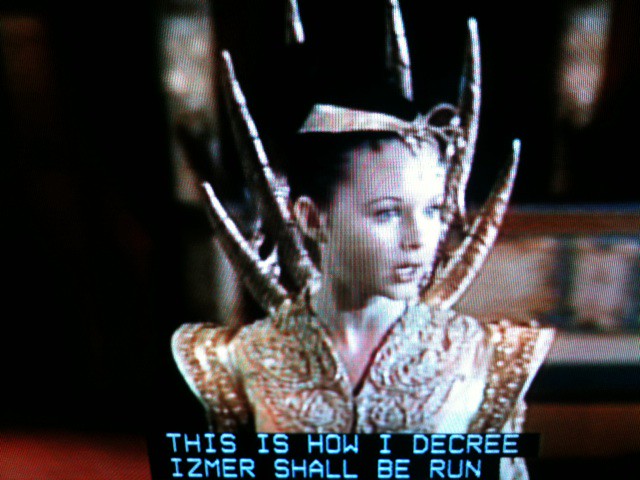In this image, which appears to be a screenshot from an older movie or TV show, we see a young girl, likely 10 to 14 years of age, dressed in a highly ornate, fantasy-themed outfit. She is of light skin with dark hair pulled back, revealing a piece of headgear in a gold and beige hue, adorned with small frills at the front. Her costume is richly decorated, featuring jeweled embellishments, beading, and possibly lace, with flared shoulders extending outwards. Remarkably, part of her costume includes six horn-like structures that protrude from her back, curving upwards and towards the camera, resembling intricate, root-like spikes. The girl is facing forward, but her head is turned to the right, showing her partially open mouth and visible teeth. The background is a blur of blue, golden, and white tones, with the lower-left corner hinting at a red carpet, and to the right, a faint light tan and gold wall. At the bottom of the image, against a black border, blueprints the subtitle: "This is how I decree Izmir shall be run," with "Izmir" spelled I-Z-M-E-R. The entire scene suggests a moment of declaration or authority within a fantastical narrative.